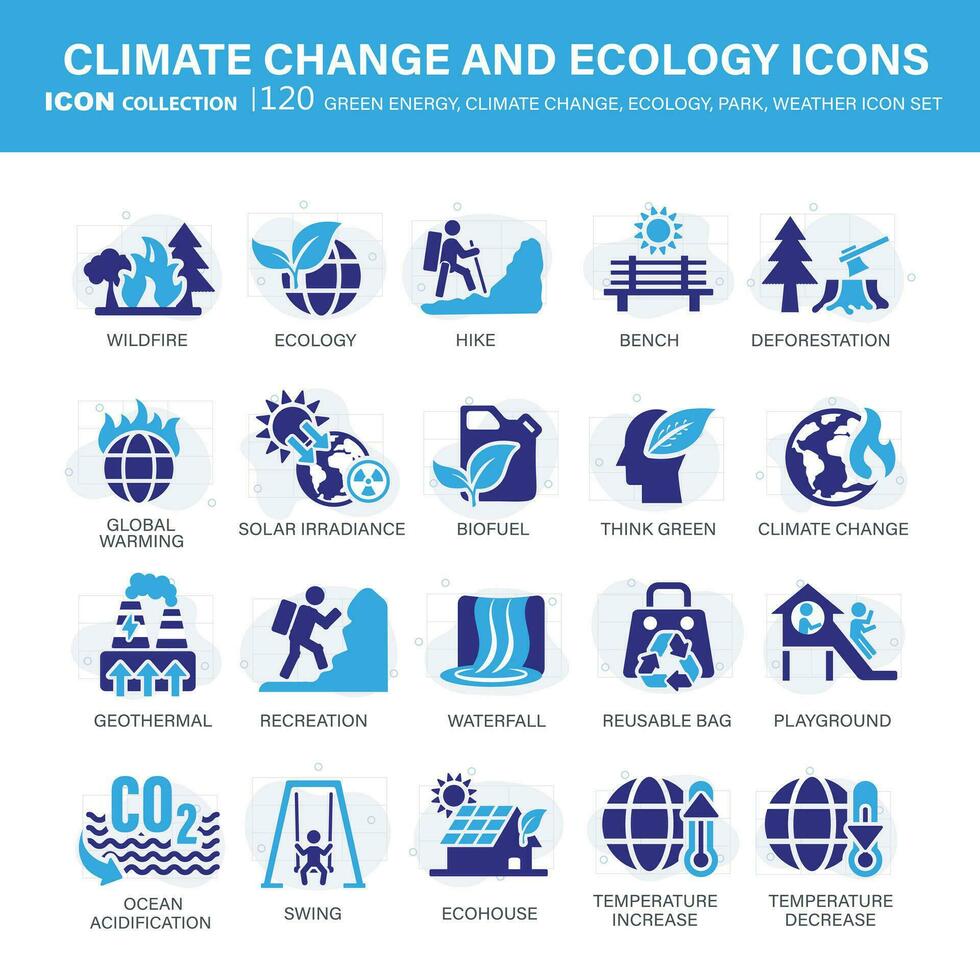The poster entitled "Climate Change and Ecology Icons" features a collection of 120 green energy, climate change, ecology, park, and weather icons on a white background with a light to dark blue gradient. The title is prominently displayed in a blue banner with white, all-capital letters. Below the title, the text reads "Icon Collection, 120 Green Energy, Climate Change, Ecology, Park, Weather Icons Set."

The icons are organized into four rows, each containing five distinct icons. The first row includes: Wildfire (a fire icon), Ecology, Hike (a figure hiking up a mountain), Bench (a bench with the sun above), and Deforestation (a tree trunk with an axe and a tree). The second row displays: Global Warming (a burning Earth), Solar Irradiance (the sun emitting rays toward Earth), Biofuel (a fuel can with a plant leaf), Think Green (a head with a green leaf on top), and Climate Change (another burning Earth depiction). 

In the third row, there are icons for: Geothermal (plants with arrows pointing up), Recreation (a hiker without a stick), Waterfall (a waterfall depiction), Reusable Bag (a bag with a recyclable symbol), and Playground (a house with a slide and a child). The fourth and final row features: Ocean Acidification (CO2 and water molecules), Swing (a child on a swing), Eco House (a house with solar panels and a green leaf), Temperature Increase (an Earth with a thermometer pointing up), and Temperature Decrease (an Earth with a thermometer pointing down).

All icons share a color palette ranging from light blue to dark blue.